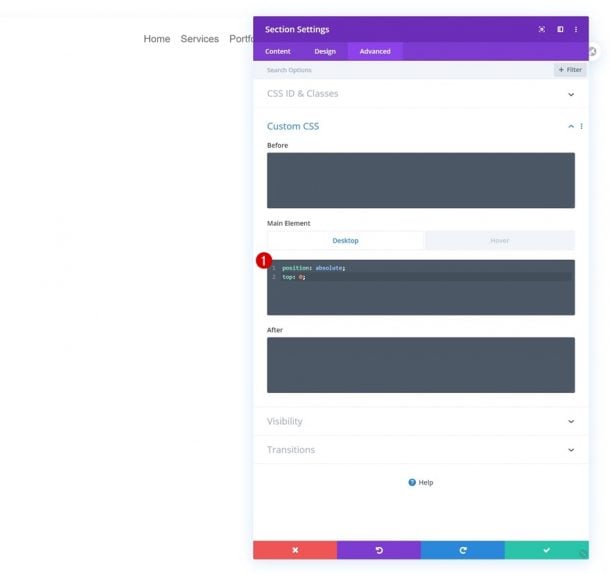The image is a screen capture of a website interface, showcasing an overlaying pop-up window. In the background, the website displays a white background with black sub-menu text. The sub-menu includes partially visible items such as "Home," "Services," and a truncated word "Portfolio."

Overlaying this view is a prominent purple banner atop the pop-up window, featuring white text that reads "Section Settings." Below this, the window is segmented into tabs labeled "Content," "Design," and "Advanced," with the "Advanced" tab being currently active. Within this tab, the interface presents options for "CSS ID and Classes," indicated by a pull-down arrow, and a section for "Custom CSS" highlighted in blue.

Further down, the "Advanced" tab includes a series of gray text boxes labeled "Before," "Main Element (Desktop)," and an undistinguishably blurry label. The word "Desktop" is rendered in teal, and the gray box contains text in green, blue, and red, accompanied by a red and white number one icon. The "After" box features similar gray text fields.

Below these boxes, there are two menus labeled "Visibility" and "Transitions," each with a down arrow for expanding options. Besides these, a blue circle icon labeled "Help" is visible.

At the bottom of the pop-up window, there are several colored buttons with white icons: a salmon-colored button with an "X," a purple back arrow, a blue forward arrow, and a teal-green button with a check mark. There are no other notable elements in the image.